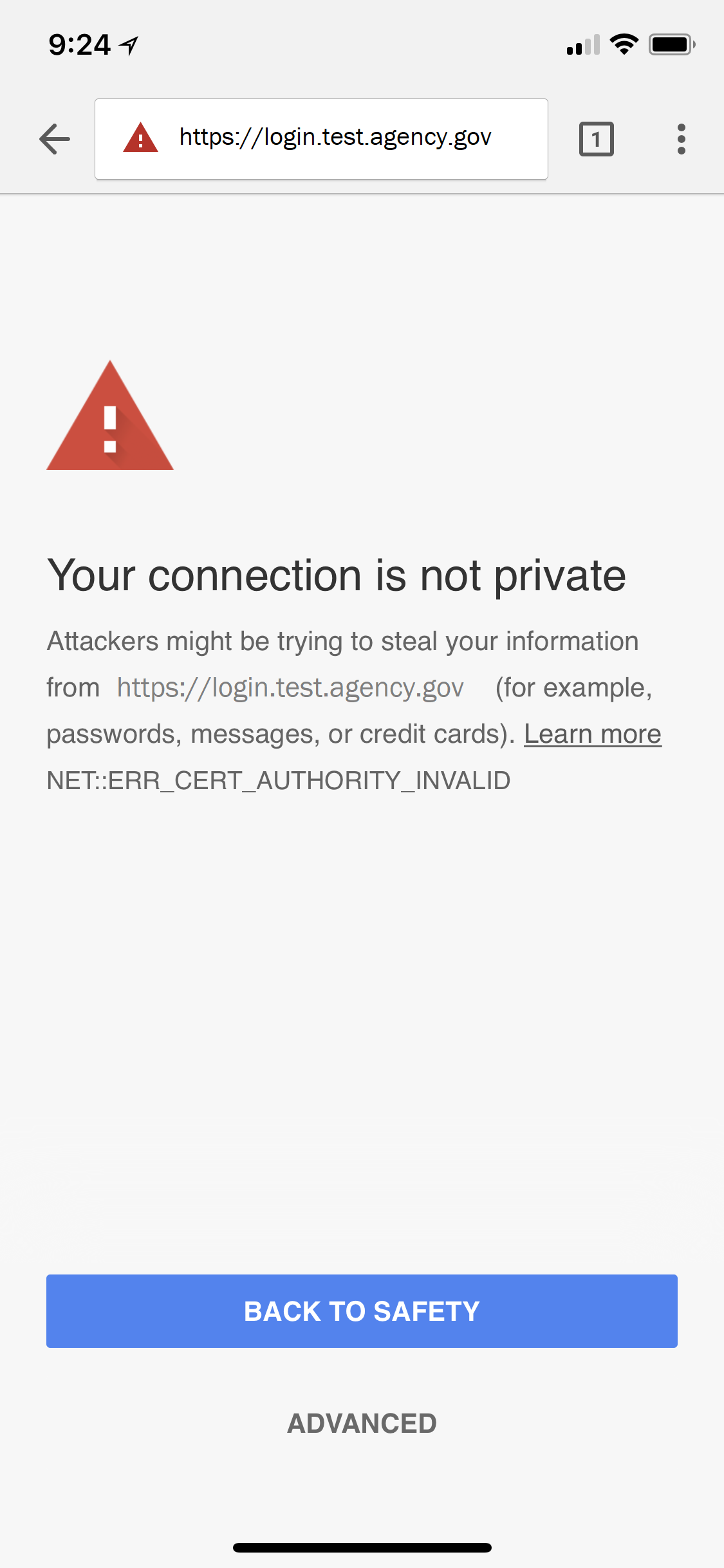The image captures a screenshot taken from a tablet or smartphone displaying a web page with a dark gray background. 

In the top-left corner, there's a "924" icon accompanied by a pointer or airplane symbol. On the top-right, there's a cell phone icon indicating a 2 out of 4 signal strength, a fully connected Wi-Fi symbol, and a fully charged battery icon.

On the left-hand side of the screen, a black arrow points towards a white rectangle featuring a red caution triangle with a white exclamation mark. Below this, a URL is displayed in black text: "https://login.test.agency.gov." 

Outside this rectangle, there is a black square with a black border that contains a black "1" and three black ellipses.

Centrally positioned on the screen, a red triangle with a white exclamation mark is superimposed against the gray background. Below it, bold black text announces, "Your connection is not private." In regular black text beneath this, a warning reads: "Attackers might be trying to steal your information from https://login.test.agency.gov." This is followed by an example in parentheses: "(for example, passwords, messages, or credit cards)."

Further down, bold black underlined text invites users to "Learn more." Below this is the error message in black text: "NET::ERR_CERT_AUTHORITY_INVALID."

A solid dark blue rectangular button with bold black text inside prompts users to return "Back to safety." Following this, there is an "ADVANCED" option in all caps black text.

The image concludes with a black navigation bezel at the bottom of the screen.